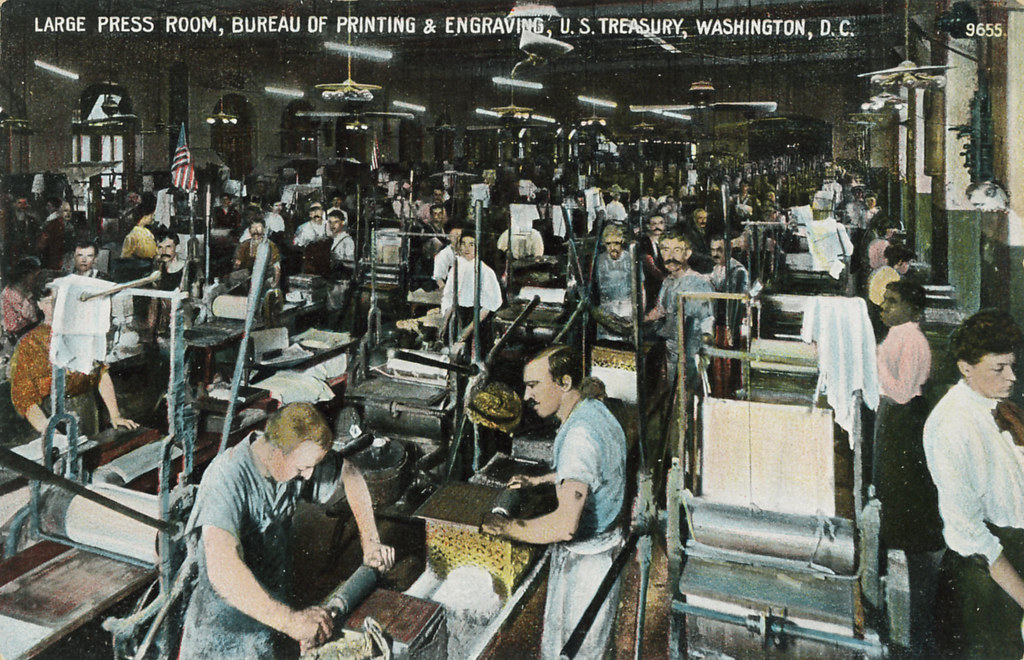This detailed painting, titled "Large Press Room, Bureau of Printing and Engraving, U.S. Treasury, Washington, D.C., 9655," offers a vivid depiction of a bustling factory interior, seemingly from the 1950s or 60s. The expansive room is filled with numerous machines, with a diverse group of approximately 150 men and women, all deeply engaged in their tasks of handling pressing and engraving machines. The workers are uniformly dressed in light blue or white shirts, contributing to a cohesive visual. Bright tube lights hang from the ceiling, illuminating the green-paneled lower walls and white upper walls with a crisp, white light. The painting captures not only the industrious atmosphere of the factory but also the historical significance of its function in the U.S. Treasury, hinting at the production of important legal documents or currency. The image is rendered in a somewhat grainy texture, further emphasizing its historical context and the meticulous labor depicted.